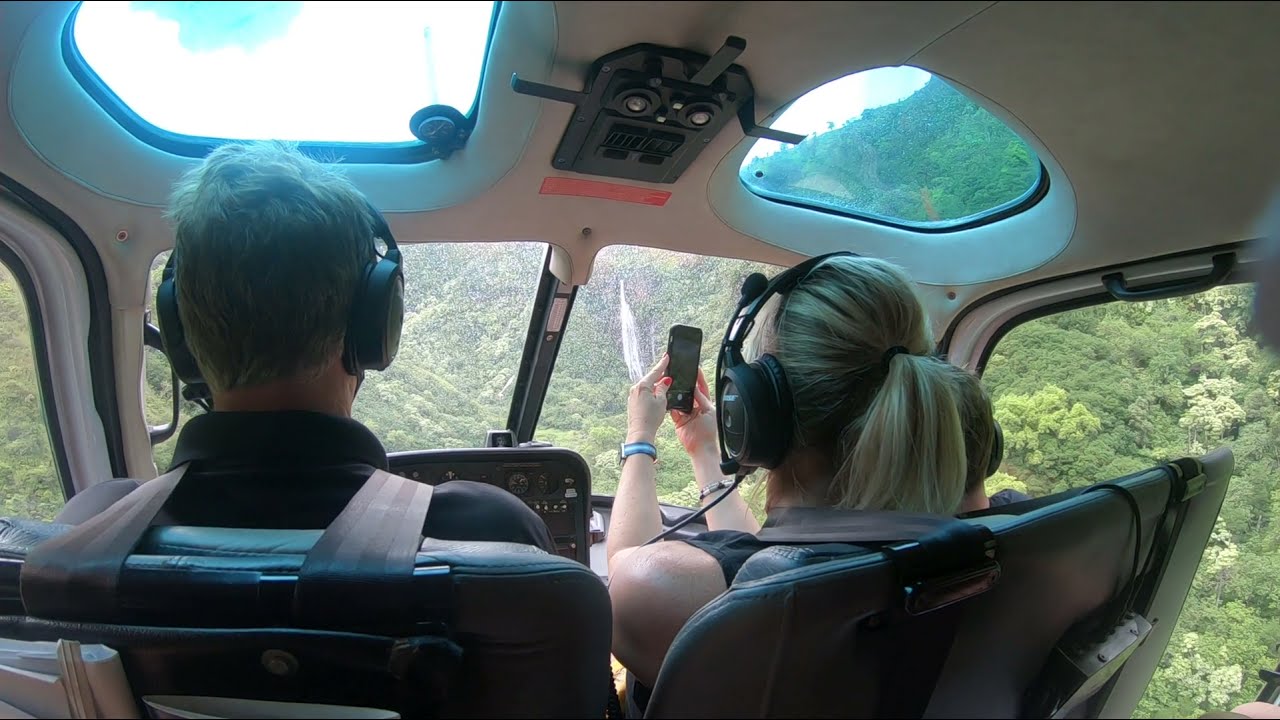The photograph captures a detailed scene likely from the backseat of a small plane or helicopter, showing a view inside the cockpit. In this horizontally oriented image, two individuals are seated in front, each wearing large black headphones and secured with harness-style seatbelts. The individual on the left, presumably the pilot, has short, slightly dirty blonde or light brown hair and is wearing a black polo shirt with a visible collar. To the right is a woman with blonde hair pulled back in a ponytail, wearing a black top, with her red-polished nails and wristwatch clearly visible on her left wrist. She holds her phone up, aiming it forward as if taking a picture through the front windshield.

In front of the pilot, parts of the control panel are visible. Both individuals are surrounded by windows; two side windows, front windows, and skylights above them. Through these windows, the outside view reveals a scenic expanse of green hills and forests, with distant mountains framing the scene. In the top left skylight, patches of blue sky and white clouds are visible, enhancing the sense of altitude and movement through a picturesque valley landscape.